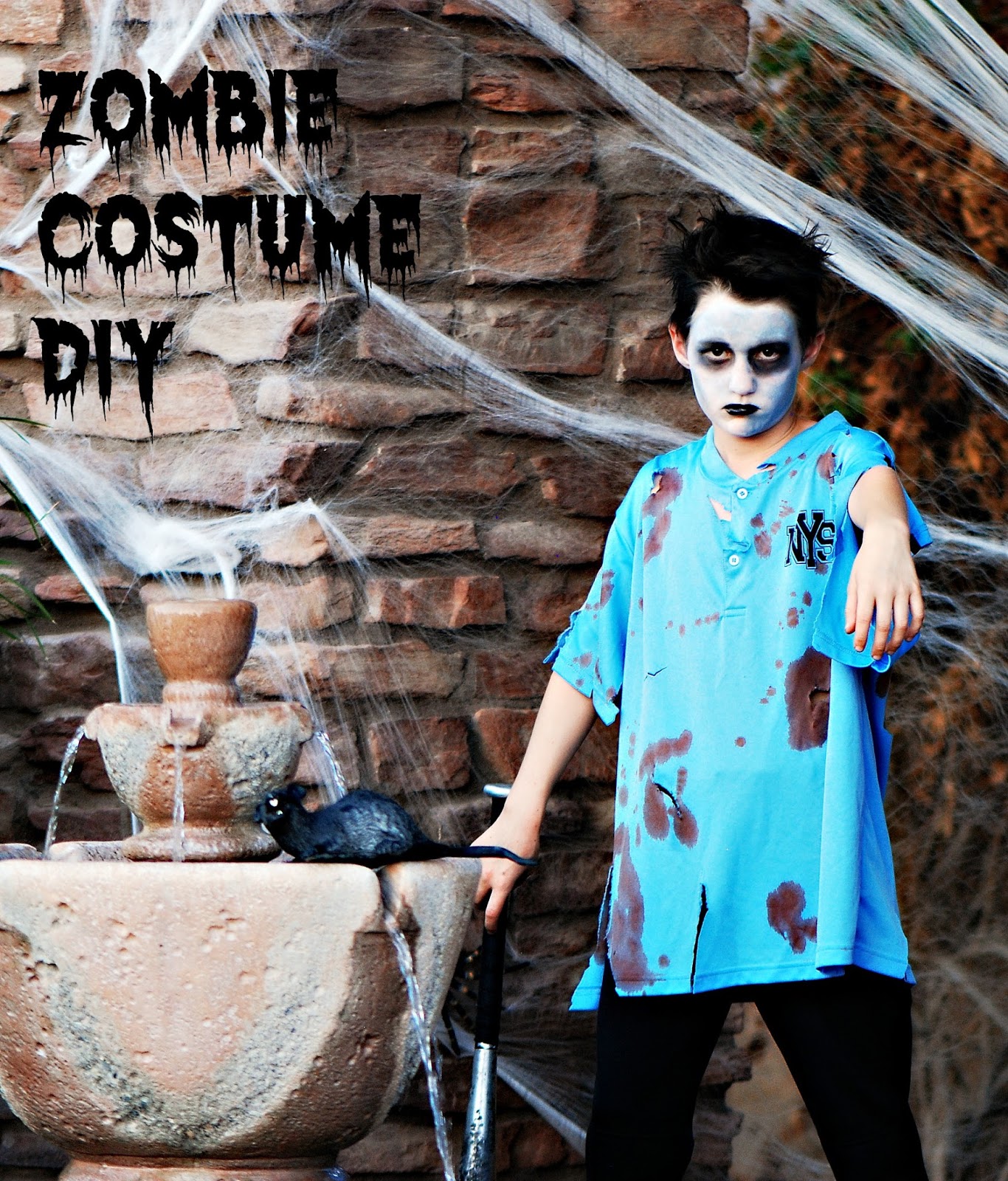In this photograph, a young boy, roughly 10 years old, is dressed as a zombie. He stands before a backdrop of a brick wall draped with cobwebs, directly facing the camera with an intense gaze. He is adorned with white face paint, accentuated by dark black makeup around his eyes and black lipstick, and his black hair is slightly spiked. The boy is attired in a tattered blue polo shirt, featuring blood-red splotches and the letters "NYS" in black. He wears black pants and extends his left arm toward the camera, bent at the wrist, capturing the classic zombie pose. To his left, a tan and brown ceramic fountain spouts a bit of water and has a faux black rat perched on it. In the top left corner, the words "ZOMBIE COSTUME DIY" are displayed in a spooky, dripping font.